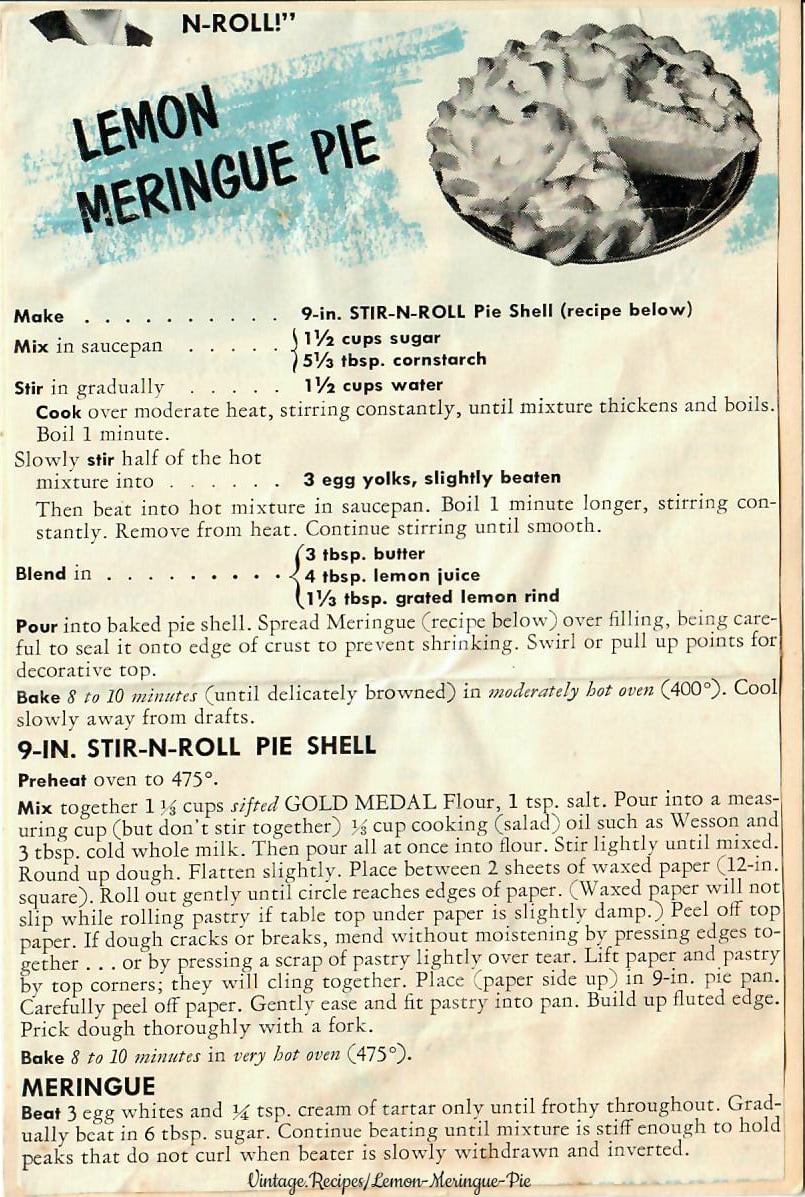This is a page, seemingly torn from an old magazine, featuring a detailed recipe for Lemon Meringue Pie. The recipe card is printed on pinkish paper and is adorned with various visuals and text that create a vintage aesthetic. In the top left corner, there's an image of a pie—possibly a roll—labeled "N-roll" in black letters. Adjacent to this, the title "Lemon Meringue Pie" is written in black letters at a slight angle against a light blue background. Below and to the right, a larger picture of a Lemon Meringue Pie with a slice taken out occupies the space.

The recipe instructions start beneath this image. They include steps such as "Make 9-inch Stir and Roll Pie Shell" and "Mix in saucepan 1½ cups sugar. Stir in gradually 1½ cups water and 5⅓ teaspoons cornstarch." The directions continue with precise instructions on combining ingredients and cooking methods, extending through roughly ten to twelve lines of text.

Towards the lower middle section, the instruction "Mix in saucepan" appears once more, followed by further details for the pie filling. Below this, in larger black letters, "Meringue" is highlighted, with subsequent lines explaining how to beat egg whites and incorporate sugar until peaks form.

Finally, at the bottom of the card in light black script, the words "Vintage Recipes Lemon Meringue Pie" are inscribed, reinforcing the nostalgic charm of this recipe page. The entire layout, with its mixed and angled texts, blue highlights, and black script, exemplifies a classic, old-fashioned cooking guide.